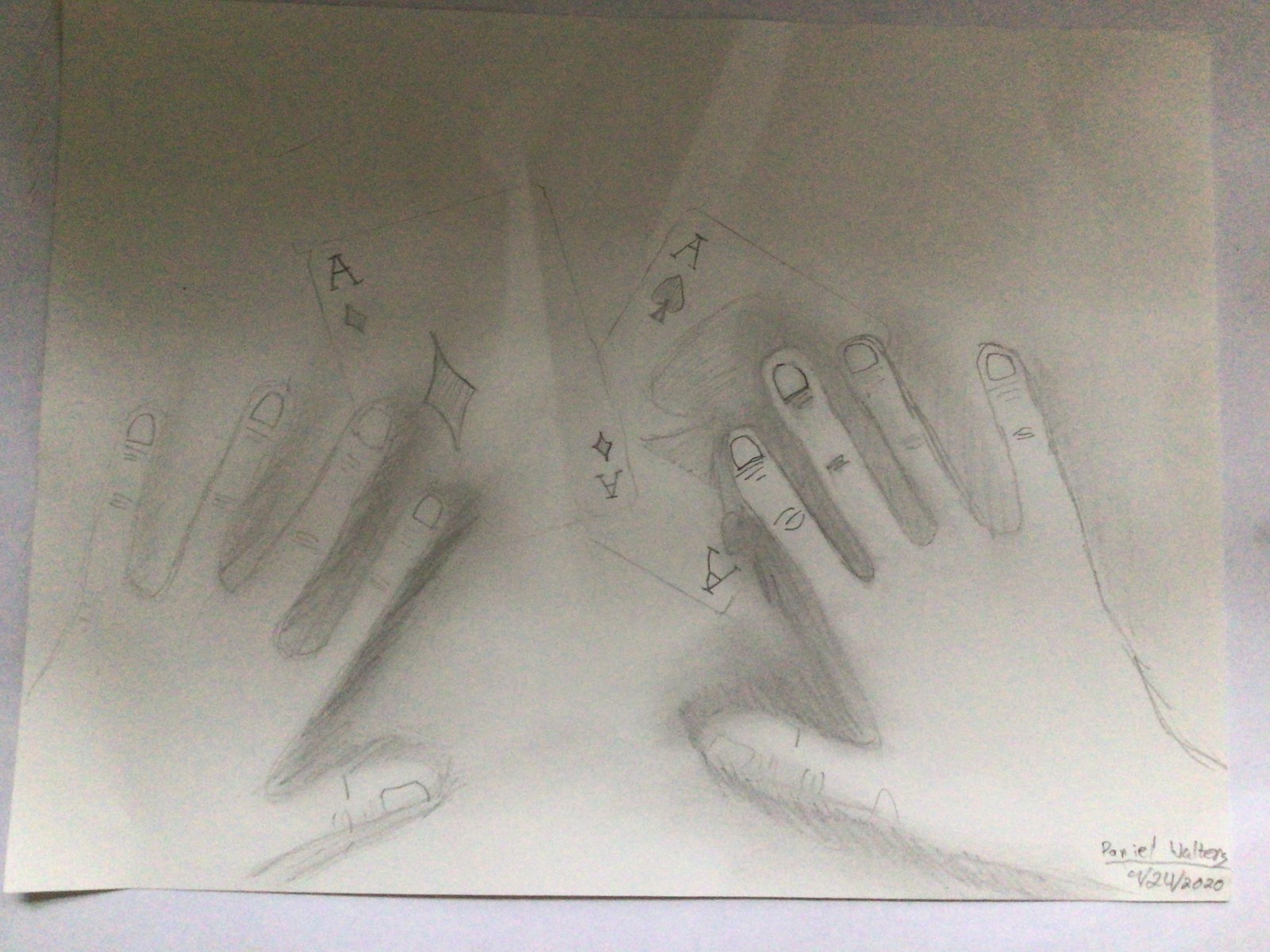This detailed hand-drawn illustration, created by Daniel Walters on April 24, 2020, is depicted on a slightly wrinkled white sheet of paper. The drawing features an artist’s portrayal of their own hands, meticulously rendered in pencil with careful attention to shading and detail. The left hand is positioned to the left of the page, while the right hand appears on the right side, both clearly showcasing contours and textures, including finely sketched knuckles and fingernails. Beneath the hands, two playing cards, specifically an ace of diamonds and an ace of clubs, are artfully placed. The background includes subtle shading, adding depth and dimension to the overall scene. Daniel Walters' signature and the date are neatly inscribed in the bottom right corner of the paper.